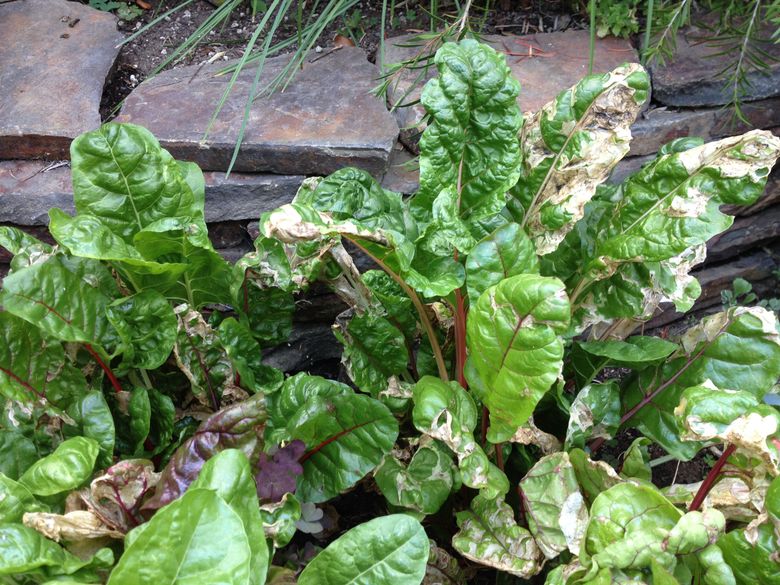This image portrays a group of outdoor rhubarb plants with large, oval-shaped green leaves that demonstrate significant signs of weathering and decay. The leaves exhibit a range of coloration from light to dark green but are marred by brown, curled edges and patches, suggesting they are wilting or dying. Some leaves appear partially eaten with irregular patches missing. At the base of the image, several plants have notably brown, entirely curled-up leaves, indicating severe distress. In the background, a stone border is visible, accentuated by a mix of brown dirt and tufts of decorative grass, along with a few other plants that might be weeds or rosemary, contributing to the rustic garden setting.